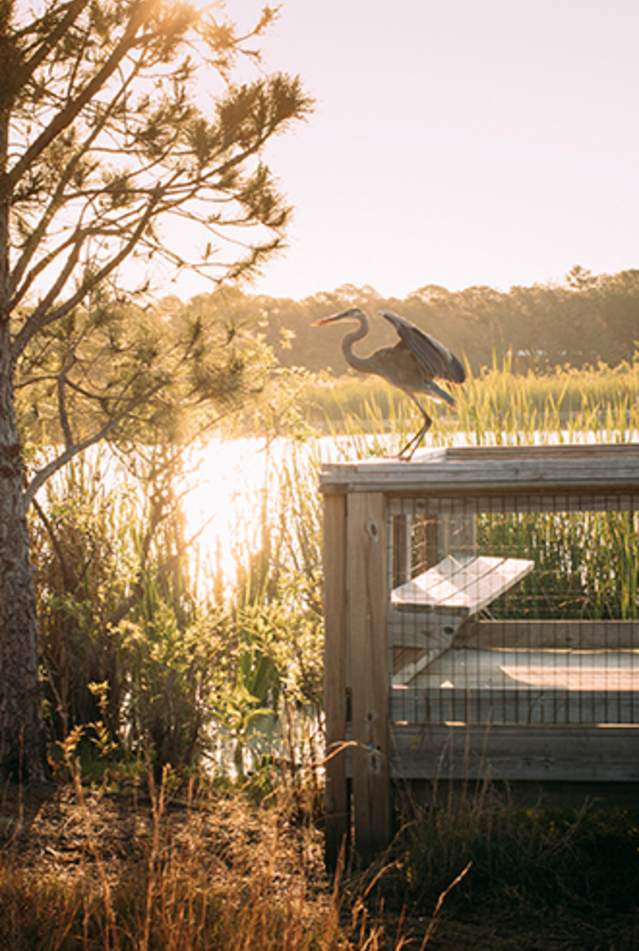In the image, a serene nature scene unfolds around sunset in a modern park. The sky, painted with the dimming hues of the setting sun, casts a reflective glow on a large body of water that stretches across the background. The water is bordered by patches of dark brown soil and grass, with unique weeds and sparse vegetation adding texture to the landscape. To the left, there's a tree with branches and leaves extending towards the top right of the frame.

In the foreground, a wooden crate or cage sits prominently on the ground, constructed of thin black wires encasing three sides and supported by a sturdy wooden frame. Resting on top of the crate is a majestic heron, wings partially spread as if preparing to take flight or having just landed. The heron's long, thin neck gracefully arches with an orange-tipped beak pointing directly to the left. Below, its legs extend down before bending at a sharp angle. Nearby, a clean wooden bench underscores the park's well-maintained appearance.

This captivating scene balances elements of nature with the subtle touch of human-made structures, creating a harmonious blend of tranquility and observation.